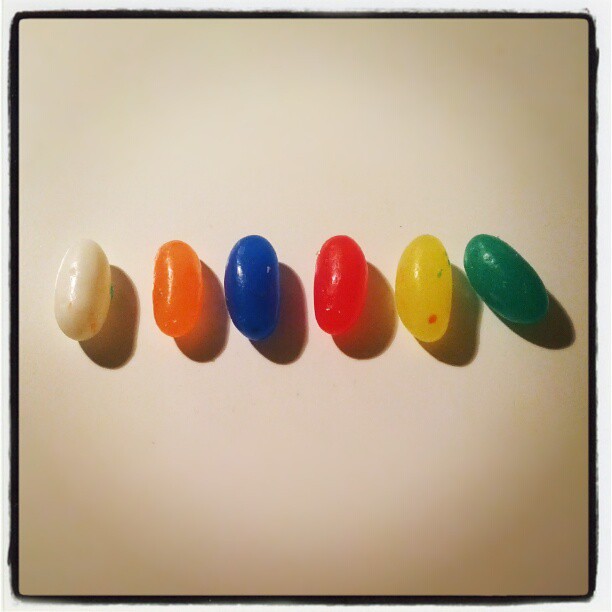This indoor color close-up photograph captures a row of six jellybeans, arranged horizontally against a smooth white background. The jellybeans, from left to right, are white, orange, blue, pink (appearing red in some descriptions), yellow, and green. Each jellybean is oval-shaped with a glossy texture that reflects light coming from the upper left, casting shadows to the lower right. The jellybeans have varying surface details, including occasional specks and dents; specifically, the white jellybean shows green and orange specks, while the yellow one has red and green specks. Notably, the green jellybean is slightly slanted to the left, unlike the others which are vertically aligned. The image is framed with a thin black border. The lighting is even and enhances the clarity of the photograph, although the lower corners of the image are subtly darker.